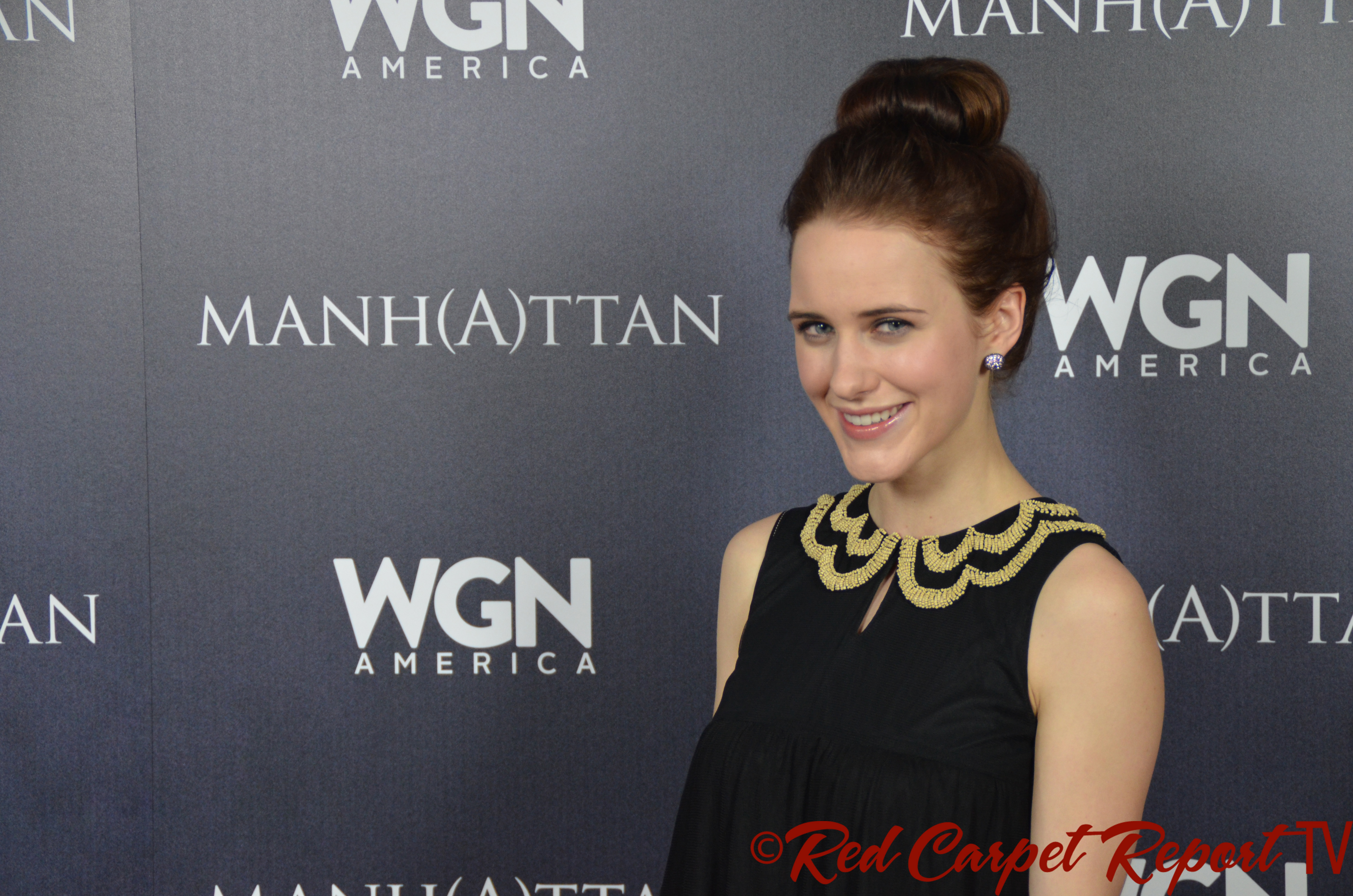The image features a white woman with dark brown hair styled in an elegant bun. The photograph captures only the left side of her face, showcasing a circular, sparkly diamond earring in her left ear. She is dressed in a sleeveless, black dress adorned with a distinctive yellow thread pattern around the neckline. The backdrop is a grey canvas filled with various advertisements, including one with the word "Manh(ATTAN)" where the 'A' is placed inside parentheses. Another prominent advertisement reads "WGN" in white capital letters, with "America" below it. In the bottom right-hand corner, the text "© Red Carpet Report TV" appears in bold red letters, indicating the source of the photo.